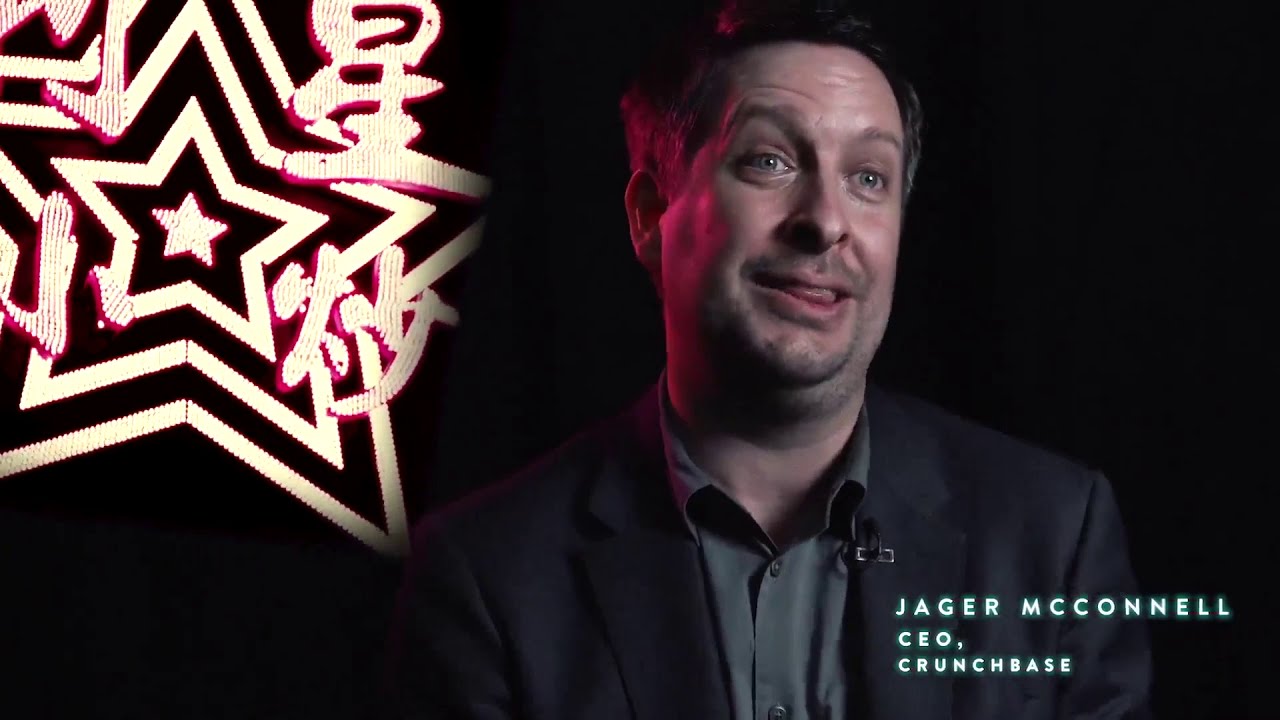This is a detailed photograph of Jager McConnell, the CEO of Crunchbase, captured in what appears to be an interview setting. He is positioned to the right in the image, with his head slightly tilted back and his tongue partially out, as if caught mid-speech. Jager McConnell's attire includes a dark gray blazer over a slightly lighter gray button-down shirt. He also sports a mic attached to his lapel. His receding hairline reveals short hair, and he has greenish-gray eyes. 

In the background, against a stark black canvas, shines a prominent neon star with intricate details: a smaller star in the center surrounded by three progressively larger outlines of stars. The lighting effect suggests a vivid, possibly neon, illumination. Notably, the image bears the designation "Jagger McConnell, CEO, Crunchbase" in the lower right corner.